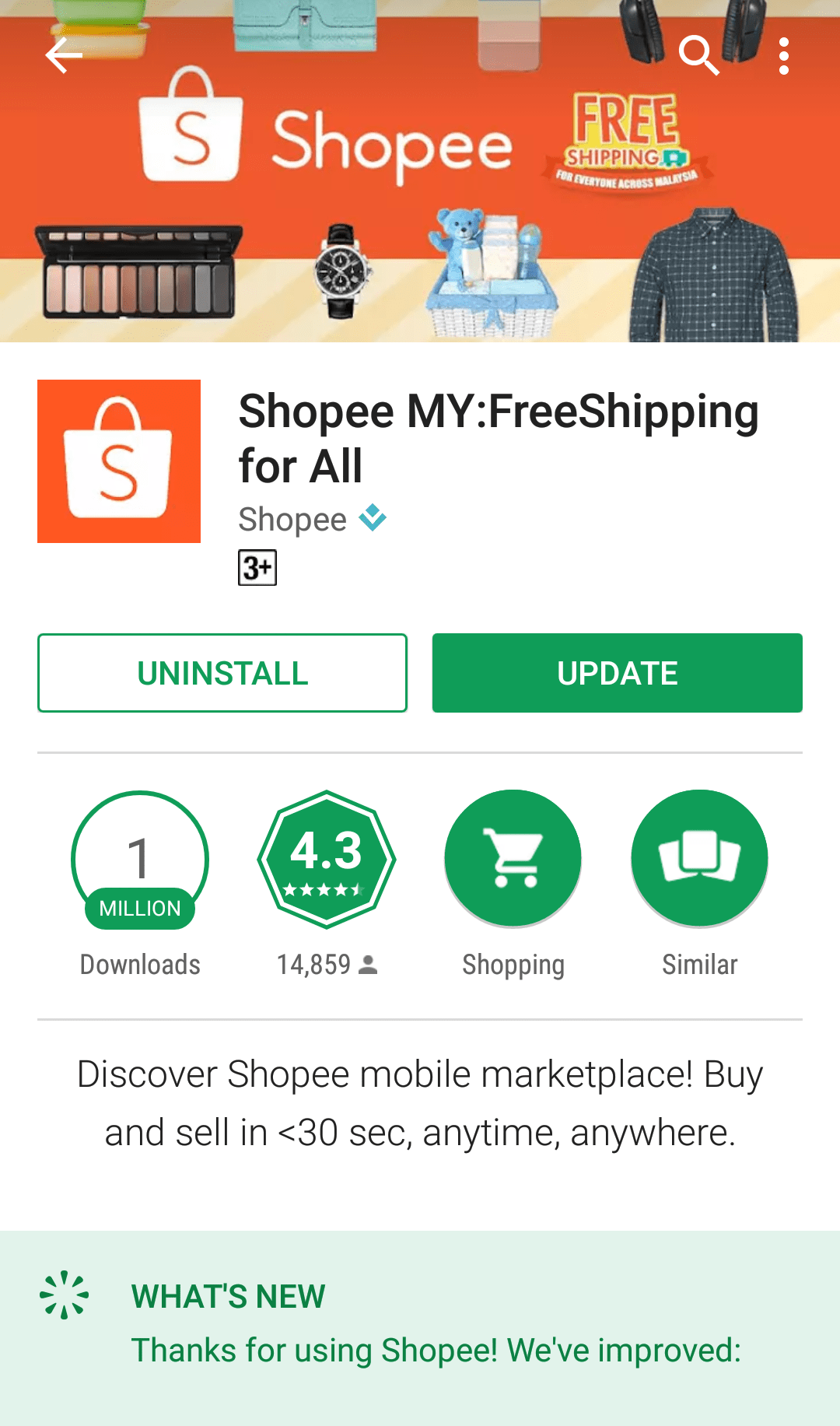This screenshot captures the interface of the Google Play Store on an Android device, specifically focusing on the "Shopee MY: Free Shipping For All" app by Shopee. The app is designed for users aged 3 and up, featuring an orange square icon with a white shopping bag and an orange 'S' in the center. 

At the top of the screen, a prominent Shopee logo banner announces free shipping for everyone across Malaysia. Below the banner, various product images are displayed, showcasing a diverse range of items such as shirts, stuffed animals, watches, and makeup.

The interface includes 'Uninstall' and 'Update' buttons in white and green, respectively. The app boasts 1 million downloads and has garnered 14,859 reviews, averaging a 4.3 out of 5 rating. It's categorized under shopping and its description reads: "Discover Shopee mobile marketplace. Buy and sell in less than 30 seconds, anytime, anywhere."

There's also a "What's New" section highlighted in light green with dark green text, stating: "Thanks for using Shopee, we've improved." The screenshot is cut off at this point. At the very top of the screen are navigation buttons, including a search button, a more options menu represented by three vertical dots, and a back button.